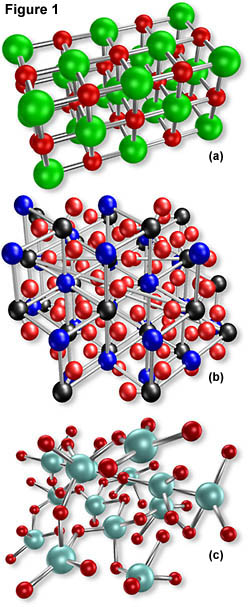The image, likely from a science textbook, showcases three distinct molecular models labeled A, B, and C. In model A, green and red molecules are connected in an organized, cubic structure, forming a three-dimensional rectangular array. Model B features blue, black, and red molecules arranged more loosely, forming smaller, potentially repetitive triangular patterns. Model C is notably chaotic, with larger teal and smaller red molecules irregularly bonded, showing no discernible organizational pattern. All three models are interconnected by white sticks representing bonds.